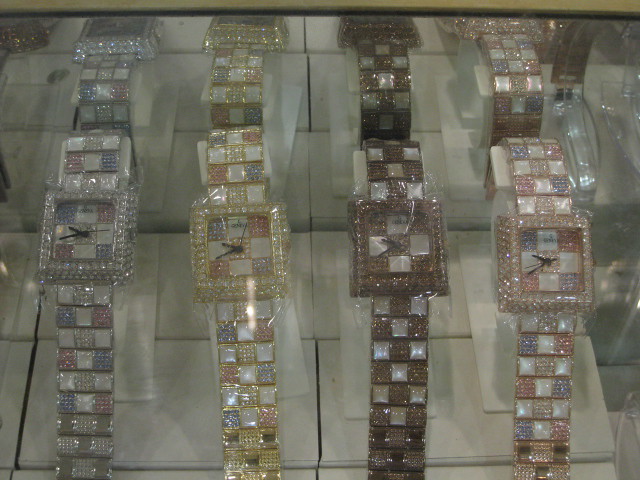This image elegantly showcases a collection of four exquisitely designed diamond watches, each uniquely crafted and exuding opulence. 

- The first watch features a luxurious sterling silver hue, adorned with meticulously cut square diamonds embedded in the watch face.
- The second watch is enveloped in a radiant yellow gold, shimmering with an array of diamonds.
- The third watch boasts a rich, dark brownish-gold finish, maintaining the same diamond-studded magnificence.
- The fourth watch gleams with a sophisticated rose gold color, also intricately decorated with diamonds around its square face.

All four watches are securely displayed within a glass showcase, ensuring their safety and illustrating their exclusive allure. The precision and detail of the diamonds around the square faces of these watches elevate their aesthetic appeal and underscore their substantial value.